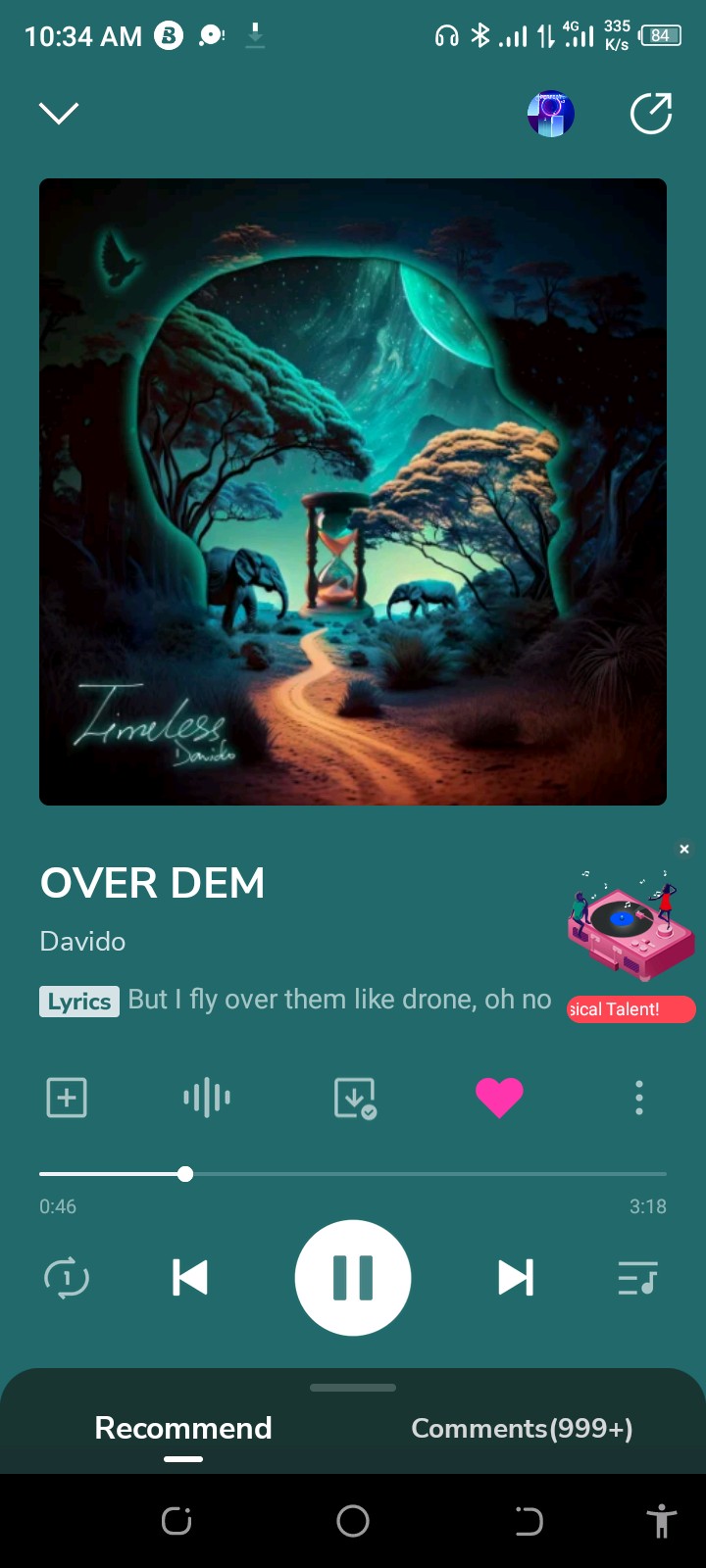The image is a screenshot captured on a smartphone, clearly indicated by the typical elements of a mobile phone's interface. At the top of the screen, the status bar showcases the current time and a series of icons on both sides. On the left, there's the time, a couple of symbols, and a download arrow with a line beneath it. On the right, there are icons for headphones, Bluetooth connectivity, cellular signal, and battery life.

The primary content of the screenshot appears to feature a music app, likely associated with an Android device, such as Google Music. The background has a dark green hue, complementing the theme of the song's artwork. The artwork itself is an artistic representation, depicting a nature-inspired, desert-like scene intersected with the silhouette of a person's head, which contains smaller elements like animals and an hourglass.

On the left side of the artwork, the word "Timeless" is inscribed, while the song title, "Over Them," is displayed prominently in white text. The artist, identified as DeVito, is mentioned right below the song title. A white bar labeled "Lyrics" features the opening line of the song: "but I fly over them like drone, oh no."

To the right, a small pop-up shows an image of a turntable with people around it and a white 'X' at the top right corner indicating the option to close this pop-up. Below this, a partially visible red bar reads "musical talent."

The lower section of the screen contains the music player control buttons, including options for pause, like, download, add to playlist, replay, next song, and previous song. At the very bottom, there are additional options to "Recommend" (highlighted in white) and "Comments."

Overall, the screenshot provides a detailed glimpse of a music playback screen on an Android device, capturing both the functional elements and the artistic presentation of the song currently playing.